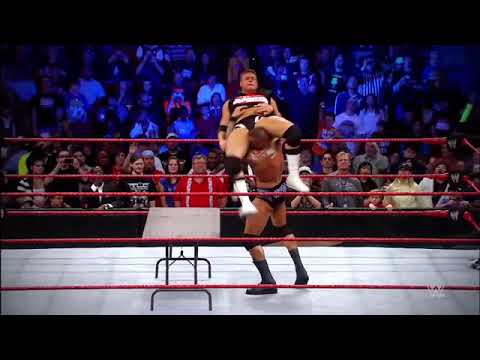The photograph captures an intense moment in a wrestling match, framed by thin black borders at the top and bottom. In the center of the white-matted ring, near a small gray folding table with black legs, one wrestler, dressed in small black bottoms, black knee straps, socks, and shoes, holds his opponent above his shoulders. The opponent is clad in black, red, and white attire, along with white boots and black knee pads. The ring is enclosed with red ropes, and beyond its bounds, a large and crowded audience is visible. The fans in the background, bathed in a blue haze, contrast with the normally lit ringside spectators, creating a dynamic atmosphere. The action within the ring suggests that the wrestler might imminently throw his opponent onto the folding table, heightening the sense of anticipation and drama.